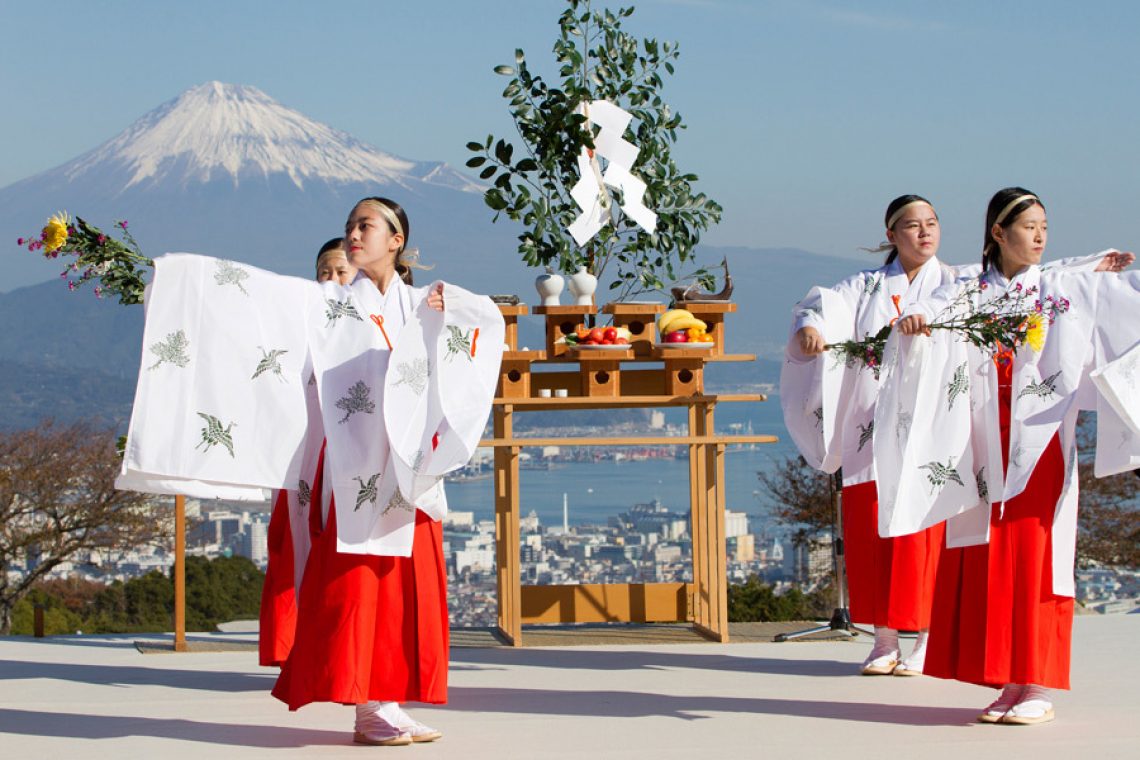The horizontal rectangular photograph captures an outdoor ceremony on a raised platform or stage. Four women, positioned two on either side of a wooden stand, are performing a traditional dance. They are dressed in traditional outfits featuring long red skirts and white coverings that drape over their arms and around their necks, adorned with designs. Each woman holds flower petals in her hands. The wooden stand in the center supports small statues, fruits, and plant stems tied with a white ribbon. The backdrop reveals several homes, a large mountain, and a bright blue sky, indicating a clear, sunlit day. The image's clarity underscores the vibrant and detailed setting of the ceremony.